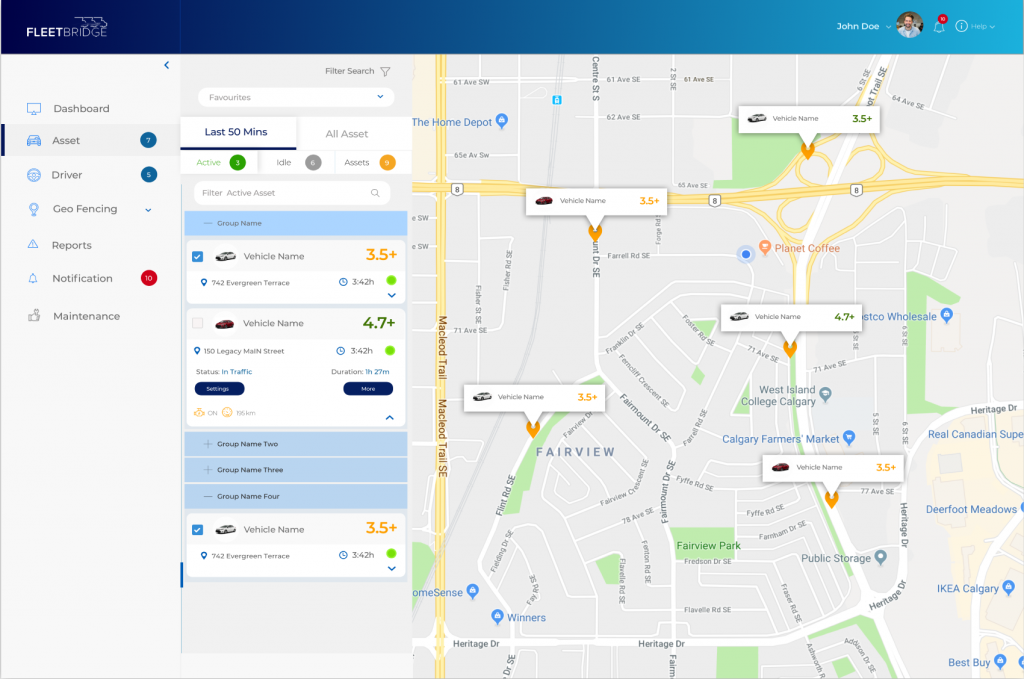This image appears to be a screenshot of a navigation and fleet management application interface. 

At the top left corner in all capital letters, it says "FLEET BRIDGE," accompanied by an icon showing the outline of three car halves stacked vertically. This label is displayed on a banner that stretches horizontally across the screen, starting from a dark blue hue on the left and gradually shifting to a lighter blue on the right.

On the far right side of this banner, the user "John Doe" is displayed, along with a profile picture of a Caucasian male. Adjacent to the profile picture, there is a notification icon containing a red circle with an unreadable number inside it, likely indicating pending alerts or messages. A small information button is also present next to the notification icon.

The left side of the screen features a vertical menu with several options: Dashboard, Assets, Drivers, Geo-fencing, Reports, Notifications, and Maintenance. Each option appears to be a clickable link for accessing different functionalities of the application.

To the immediate right of this vertical menu, there is a section displaying navigation details, labeled “Last 50 Minutes,” which includes information related to vehicle names and activities. The context suggests that the user might be tracking a fleet of vehicles.

Dominating the main area of the screen, a map shows various roads and landmarks. Notable locations on the map include Deerfoot Meadows, IKEA, Calgary, and Best Buy towards the bottom right side, while Winners is indicated on the left. Prominent roads visible on the map include Mackwood Trail and Route 8, crossing horizontally across the display. The roads and layout suggest a detailed urban area likely used for precise navigation and fleet management.